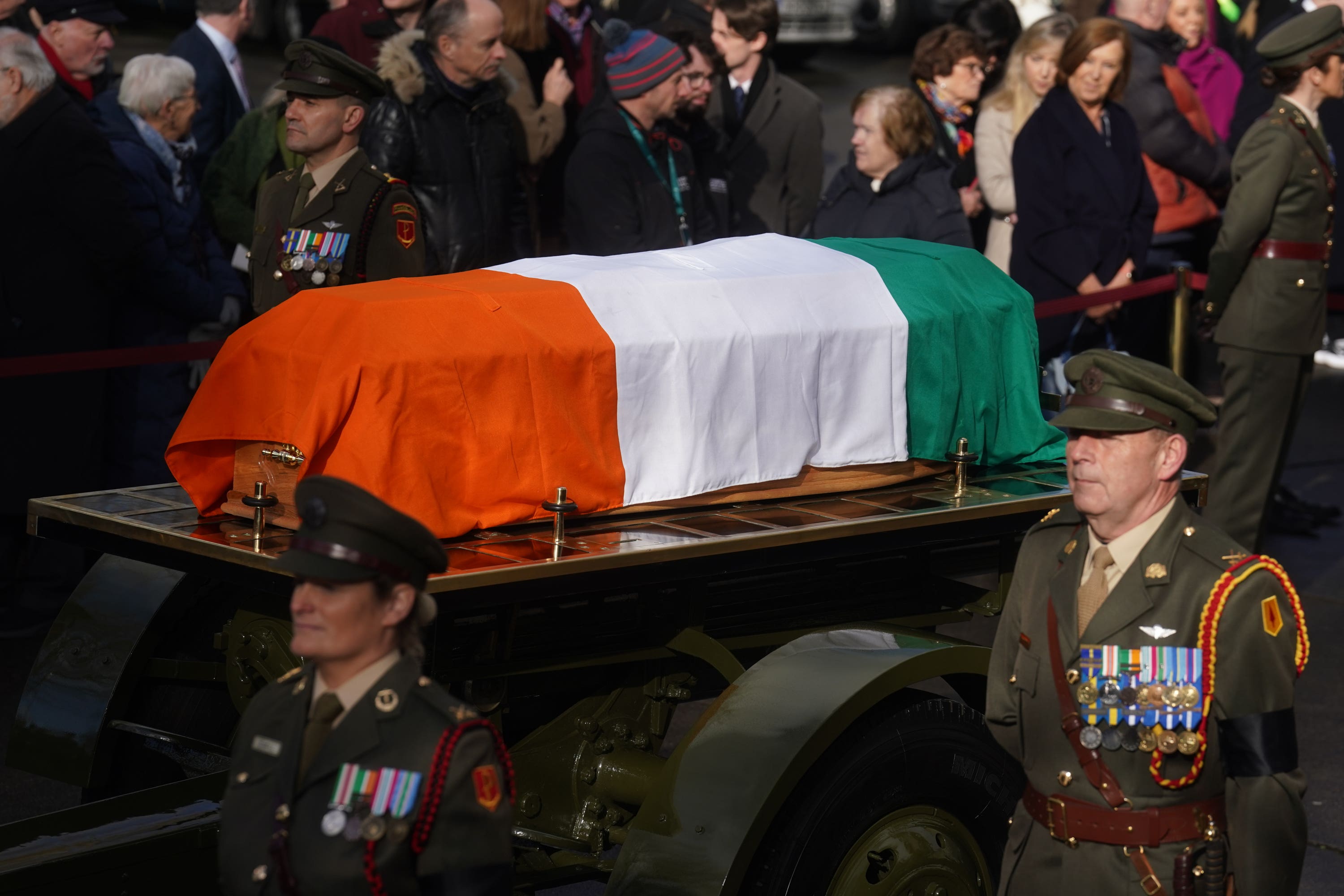The image depicts an outdoor funeral procession for a military individual or government official. The casket, draped with an Irish flag, is mounted on a piece of military equipment resembling a carriage with wheels. It is flanked by solemn military personnel dressed in green uniforms and tan ties, adorned with various medals and ribbons. One distinguished soldier stands on the right, highly decorated, while another soldier is positioned on the left, also displaying several medals. A woman in uniform stands just in front of the casket, and another woman is seen behind the casket, surveying the crowd. In the background, a crowd of onlookers, dressed in winter attire with coats and hats, stands behind a red rope barrier supported by gold posts, intently observing the solemn event. The atmosphere is one of reverence and respect.